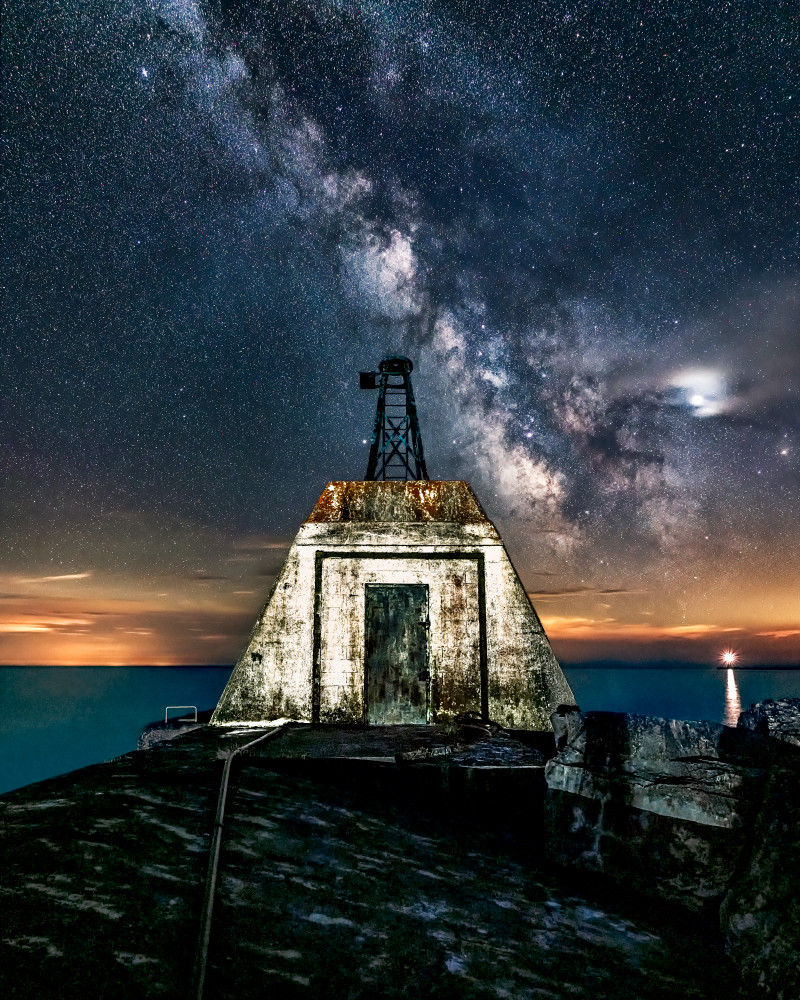The image showcases a night scene featuring a weather-beaten white building, situated in front of a dark blue ocean. The building, marked with prominent brown stains, has a black metal tower and a dark, dirt-streaked door. In front of the structure, which has a high-contrast, rusted texture, there is a stone that resembles black granite or obsidian. The horizon distinctly separates the dark, star-studded sky from the golden-orange clouds and deep blue sea. Above, a vibrant night sky is filled with thousands of stars, stretching from the top left to the center right, showing edges of the Milky Way. A bright light shines in the distance across the water, adding to the ethereal quality of the scene.